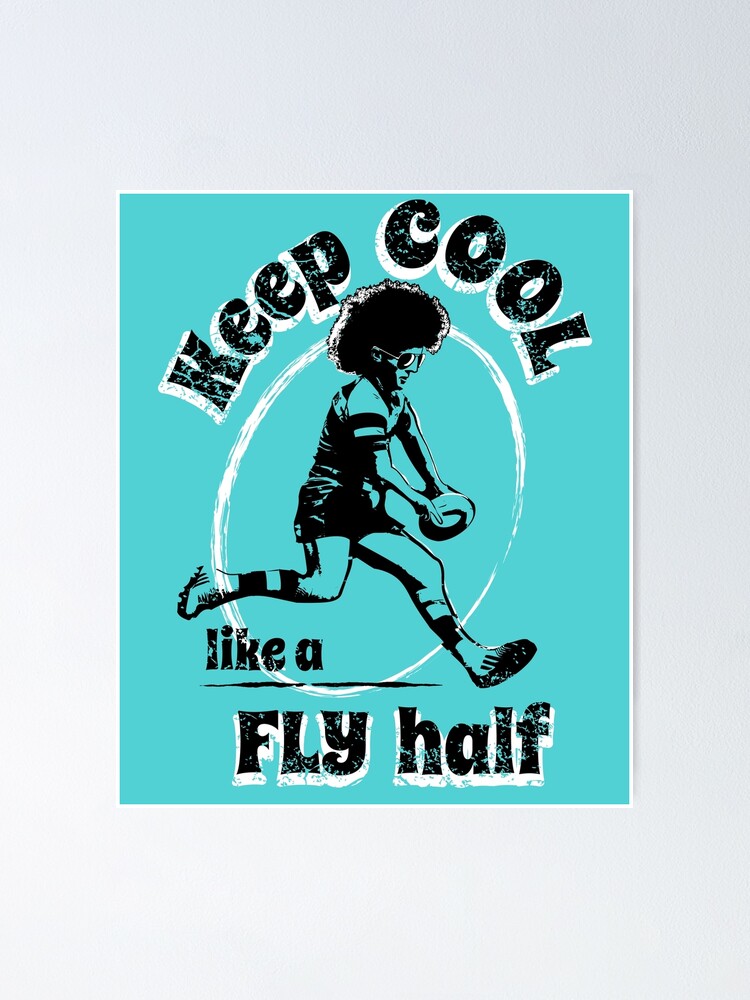The poster displays a striking image set against a turquoise or aquamarine background. Dominating the scene is a man mid-run, encircled by a white oval shape, accentuating his energetic motion. Sporting an afro and aviator sunglasses, he wears a sports jersey with distinctive stripes, short shorts, jockey socks, and Adidas cleats. Clutched in his hands, potentially prepared for a kick, is a rugby ball. The poster's text, crafted in a bold, chunky, and loopy font, proclaims, “Keep cool, like a fly half” in large black letters with a white outline. This vibrant and dynamic scene is framed against a white wall, ensuring the lively imagery and inspiring message stand out.